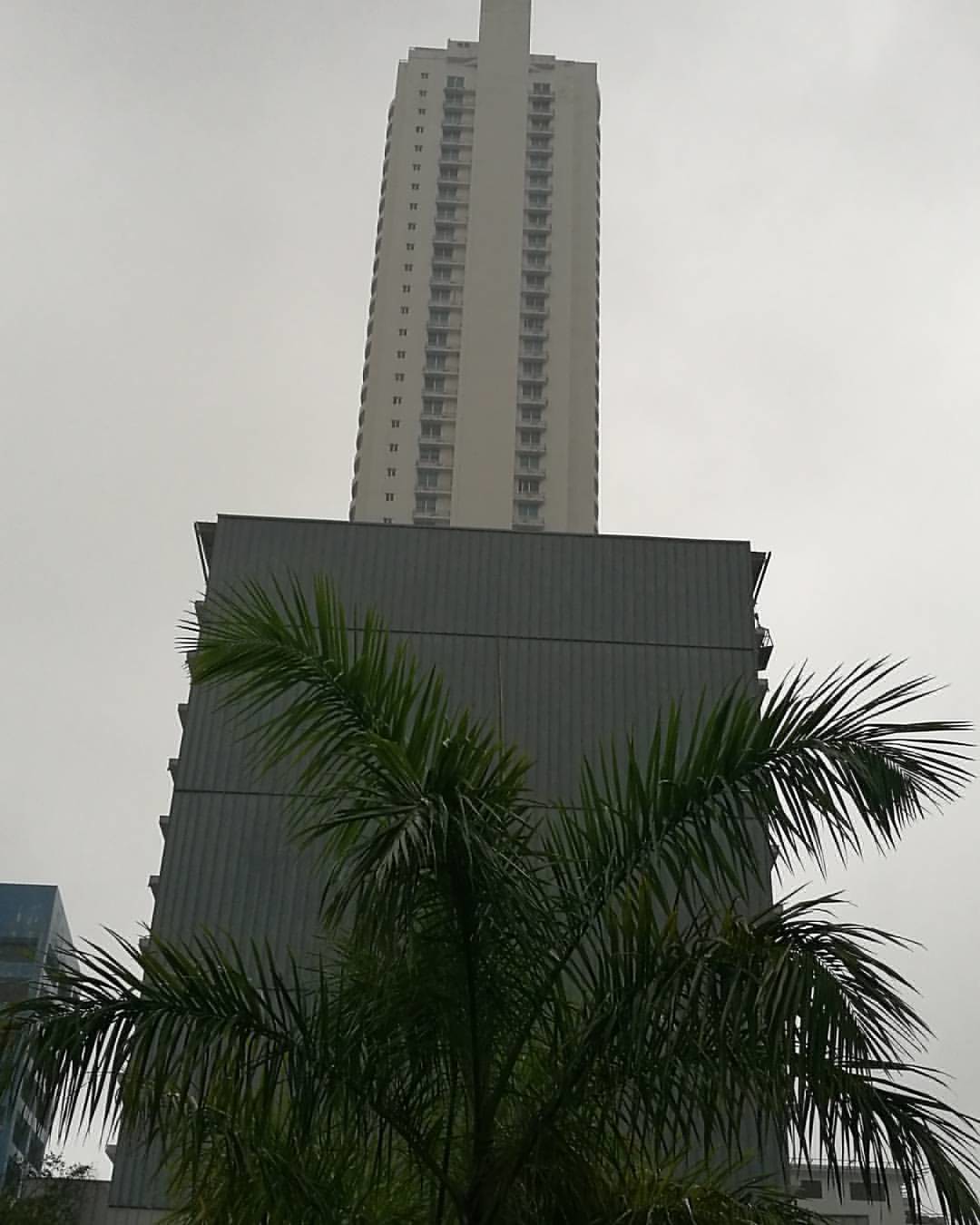The image captures a bustling urban scene dominated by a towering skyscraper, presumably around 50 stories high, that appears to be either an apartment complex or a hotel. The building features numerous balconies granting expansive views of the surrounding cityscape. To the left and right of this gray structure, additional buildings are visible, including a second prominent one at ground level, approximately 10 to 15 stories high.

At the forefront of the image stands a tall palm tree, its lush green fronds positioned about 5 to 10 feet away from the photographer, partially obscuring the view of the scene behind. The sky overhead is completely overcast, blanketed in gray clouds, casting a muted light across the landscape.

Adjacent to the main skyscraper, other buildings of varying heights and forms can be seen, contributing to the dense architectural tapestry. The foreground structure, potentially where the photo was taken from, frames the larger building and the palm tree, indicating the shot might be from a balcony or a low level looking upward.

Overall, the scene blends natural greenery with an urban skyline, framed under a cloudy sky, emphasizing the contrast between the towering modern structures and the small piece of nature in the palm tree.